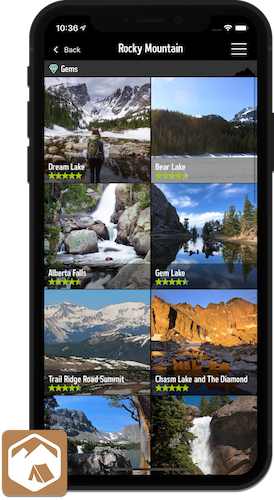In this image, we are looking at a screenshot of a black cell phone set against a white background. The cell phone is standing vertically with its screen turned on. At the top center of the screen, large, bold, white text reads "Rocky Mountain." In the upper left corner, it indicates the time as "10:36" in white text. The upper right corner shows the Wi-Fi symbol and a full battery icon. To the left of the "Rocky Mountain" text, there is a "Back" button accompanied by a left-pointing arrow.

There are eight photo images displayed on the screen, arranged in four rows with two images per row. Each image is of identical square size. The first row features images labeled "Dream Lake" and "Bear Lake." The second row contains images labeled "Alberta Falls" and "Gem Lake." In the third row, the images are labeled "Trail Ridge Road Summit" and "Chasm Lake and the Diamond." The fourth and bottom row has images without any descriptive text, leaving their subjects unidentified. In the lower left corner of the screen, there is a brown and white logo depicting a white mountain.